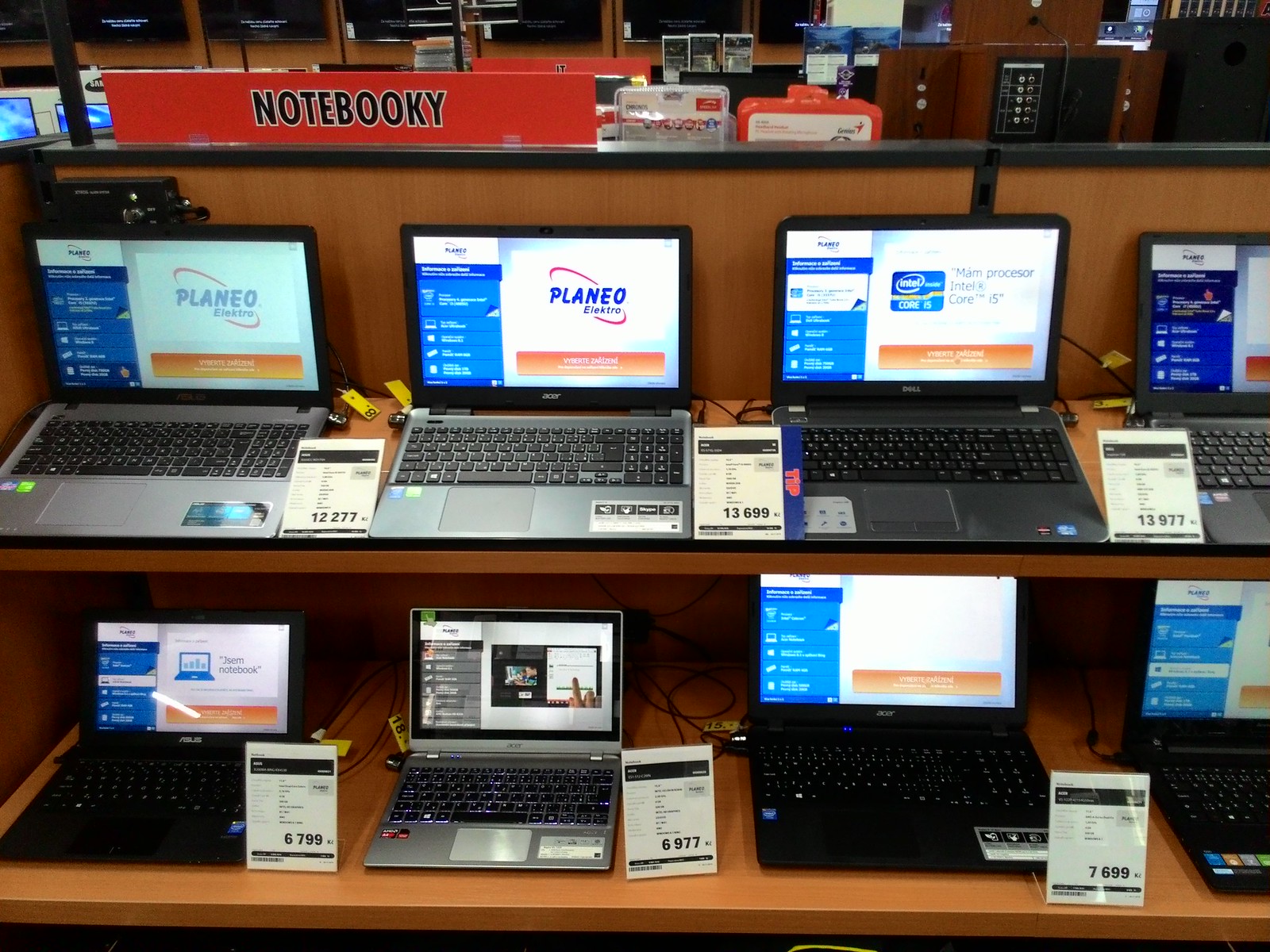The image depicts a detailed display of eight laptops inside an electronics store, likely specializing in information technology or similar products. The store's interior is visible in the background, with various other items on display. The focal point features two rows of wooden shelves, each shelf holding four laptops. The shelves themselves are a light brown wood color with black trimming. 

Above the shelves, in the top left-hand corner, there is a prominent red sign with black letters that reads "Notebookie," suggesting either the section's name or the name of the store, which seems to be non-English speaking. Each open and powered-on laptop displays varying details. On the top shelf, three laptops have screens that display the logo "Planeo Elektro." These laptops have visible price tags showing prices ranging from $12,277 to $13,977. The bottom shelf also has four open laptops with displayed screens and price tags, with slightly lower prices ranging from $6,799 to $7,699.

Of the visible laptop brands, Acer, Asus, and Dell are identifiable. The laptops appear to be a mix of newer and older models, with some smaller in size compared to others. Overall, the image suggests a diverse range of laptops available for sale in this well-organized electronics store display.